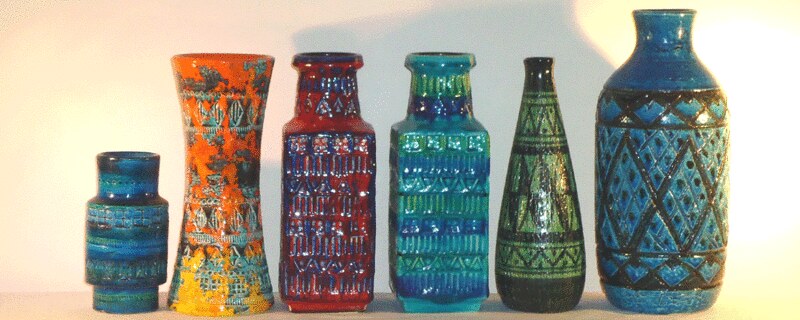This photograph features six distinct vases arranged from left to right against a white backdrop, resting on a light-colored table. The vases range in shape, size, and color, with detailed patterns enhancing their designs. 

From left to right:
1. The first vase is the shortest, about half the height of the others. It has a gear-like shape and is adorned in a mix of dark blue, light blue, green, and black.
2. The second vase is orange with yellow and black accents. It has a wide base, narrows at the center, and widens again at the top, resembling a teardrop or an hourglass.
3. The third and fourth vases share a similar shape: a square base that tapers upwards into a rounded neck and lip, reminiscent of a stout beer bottle. The third vase features a red hue with some blue accents, while the fourth sports a combination of blue and green.
4. The fifth vase is predominantly green with shades of light and dark green in a tapered shape, like a wine bottle.
5. The sixth and tallest vase is a striking blue with black patterns. It has a wide, rounded base and a narrower neck, reminiscent of a milk jug without a handle.

The vases are illuminated by a bright light source coming from the right side of the image, casting subtle shadows and highlighting their textures and colors.